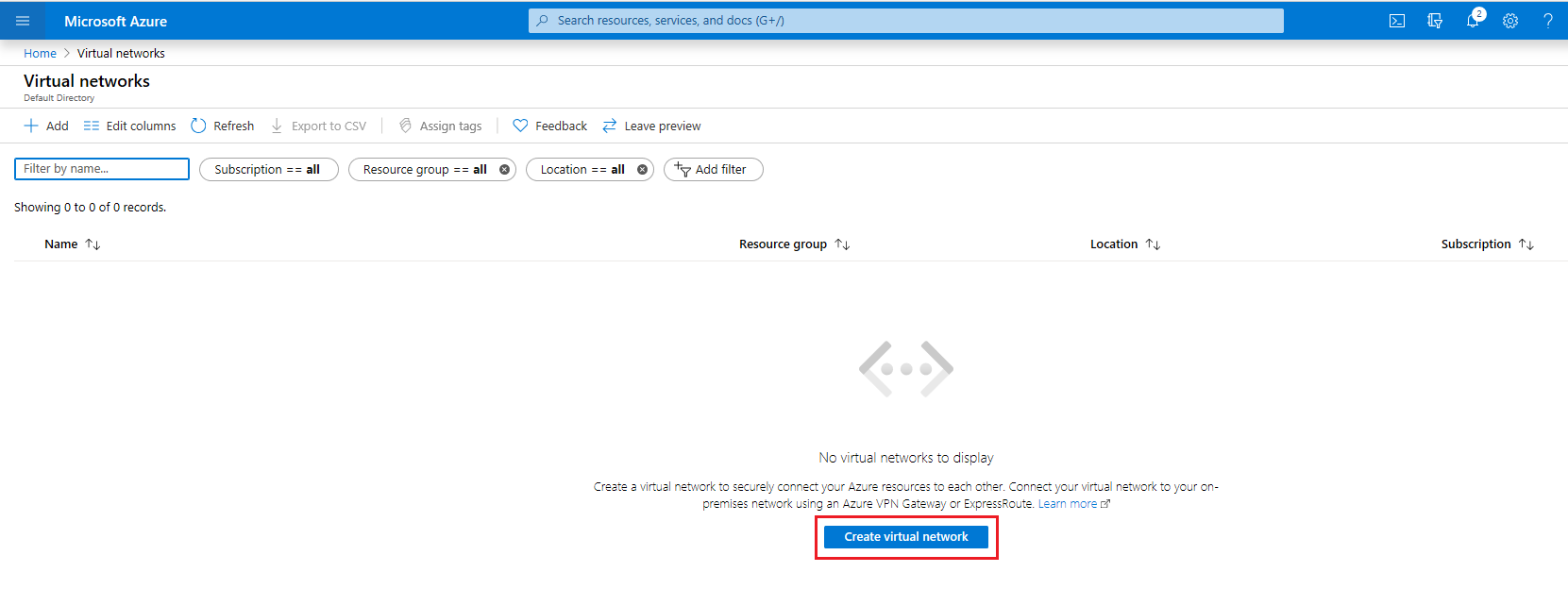In the top left of the image, the Microsoft Azure logo is prominently displayed in a mid-blue bezel. On the left side, a dark blue square contains three white lines indicating settings. Centrally within this bezel, a light blue rectangular search bar with a grey magnifying glass icon invites users to "search resources, services, and docs." This text is followed by "G+\" within parentheses. To the far right of the rectangle, back in the mid-blue bezel, there is a white square with a right-pointing arrow, an underline, a folder, a flashlight icon, and a notification bell. A white circle with the number "2" inside indicates two notifications. Additionally, there is a gear icon and a question mark icon.

On the left-hand side, two buttons are displayed: the first button, "Home," is selected and shown in blue with a grey arrow next to it. Beneath it, "Virtual Networks" is presented in bold black text, with "default directory" in grey. Various buttons are available: a blue button labeled "Add" in black, "Edit Columns" next to a refresh symbol also in blue, and next to these, a grey, faded-out arrow pointing down with "Export to CSV" in all caps. The area also contains three close-packed tags labeled "Assign tags," which are greyed out. 

A blue heart icon identifies the "Feedback" tab, which displays "Feedback" in black. Next to it, there are directional blue arrows and "Leave preview" in black text. A dark blue-bordered rectangle underneath includes grey text "Filter by name" followed by three ellipses. Various filter options are presented as black text within oval buttons. "Subscription" and "Resource group" each have "==" and bold "all" indicators, while "Location" also includes the same formatting, and an additional "remove" icon featuring a black circle with a white "X" is present.

Displayed in bold text, the filter results header includes "Name," "Resource Group," "Location," and "Subscription" each with respective up and down arrows for sorting. In the central panel, a greater than or less than symbol with three ellipses indicates no virtual networks are currently displayed. A call-to-action message prompts users to create a virtual network for securely connecting Azure resources and provides an option to connect to an on-premises network via VPN gateway or Express Route. An actionable "Learn More" hyperlink in blue text is featured along with a square icon, indicating navigation to another page. At the bottom, a dark blue rectangular button with white text offers the option to "Create virtual network," highlighted with a red rectangle to guide the user.